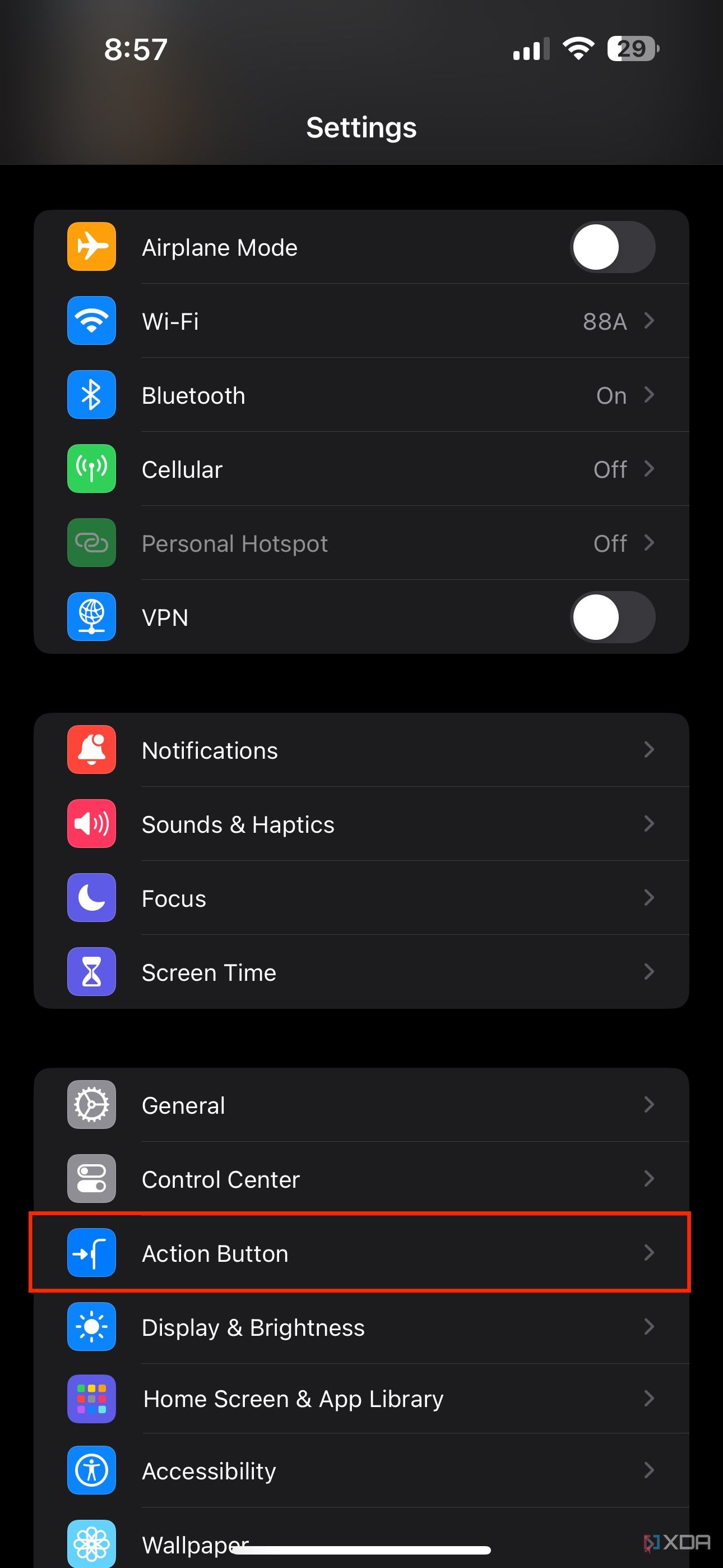The image displays a black background, predominantly in the top left corner. In white text, the time shown is 8:51. The screen also indicates that the device has decent cellular service with three out of four reception bars filled, excellent Wi-Fi connectivity with all bars full, and a battery level currently at 29%.

Centered on the screen is the word "Settings," followed by a series of options within rectangular boxes. The first box contains "Airplane Mode," displayed in white text. The next boxes list "Wi-Fi," "Bluetooth," "Cellular," "Personal Hotspot," and "VPN." Adjacent to "Airplane Mode" is a toggle switch, with the left side white (indicating 'off') and the right side gray.

Further down, additional options appear: "Notifications" at the top, followed by "Sounds & Haptics," "Focus," and "Screen Time," each accompanied by an arrow pointing to the right, suggesting further settings available. 

In the final section, "General" is listed first, followed by "Action Button," which is distinctly bordered in red, "Display & Brightness," "Home Screen & App Screen," "Accessibility," and "Wallpaper," each also featuring a right-pointing arrow for additional selections.